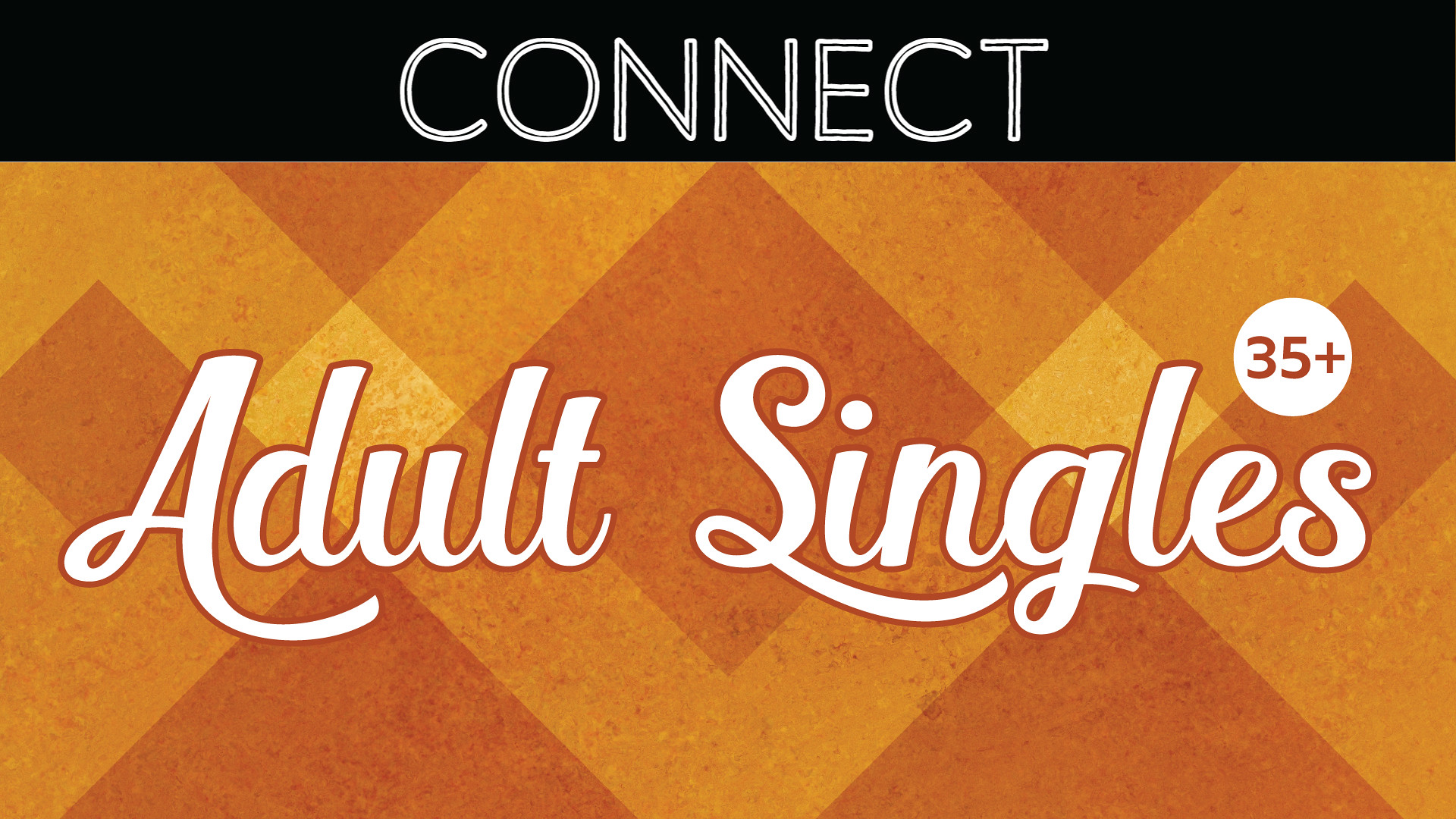The image is a long rectangular sign with a simplistic yet striking design. At the top, there's a black bar featuring the word "Connect" in bold white letters. Below this, the background transitions into a plaid pattern made up of various shades of orange, from light to dark, creating a geometric look. Centered on this orange backdrop, the phrase "Adult Singles" appears in a white cursive font, accentuated with a dark orange outline. Near the word "Singles," there is a small white circle containing the text "35+" in bold letters. The overall message promotes connecting adult singles aged 35 and over, likely indicating a dating service or event.